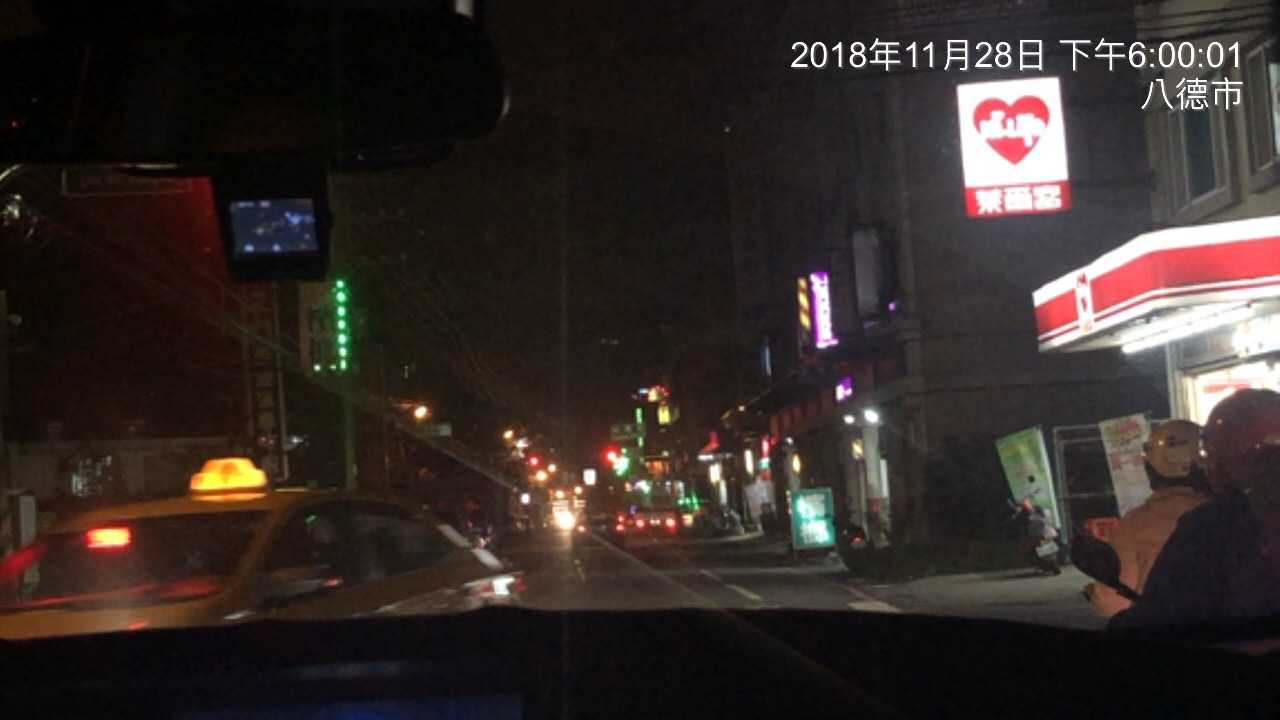The rectangular image, with its long side oriented horizontally, is a nighttime photograph taken from inside a dimly lit vehicle. The view through the front windshield is somewhat marred by reflections and streaks of light. The date "2018-11-28" and the time "6:00:01," flanked by Asian characters, are displayed at the top right, suggesting an early morning or evening hour.

In the foreground, part of the vehicle’s dark dashboard is visible, with minimal discernible details other than a flat, tiny video screen on the driver's side visor. To the left, a taxi, identifiable by its yellow rooftop marker, is moving in the opposite direction. 

On the right side of the street, two helmeted individuals ride either a moped or a scooter. Below a red sign featuring a heart and Japanese text, sits a convenience store adorned in a matching red and white color scheme. 

The bustling city street is lined with buildings on either side, ablaze with bright neon signs and various lights. Parked motorcycles are noticeable on the right, while multiple cars fill the middle of the street, halting under red traffic lights, their brake lights glowing. This scene captures an area that seems lively with numerous shops, restaurants, and stores, illustrating a typical urban hotspot.